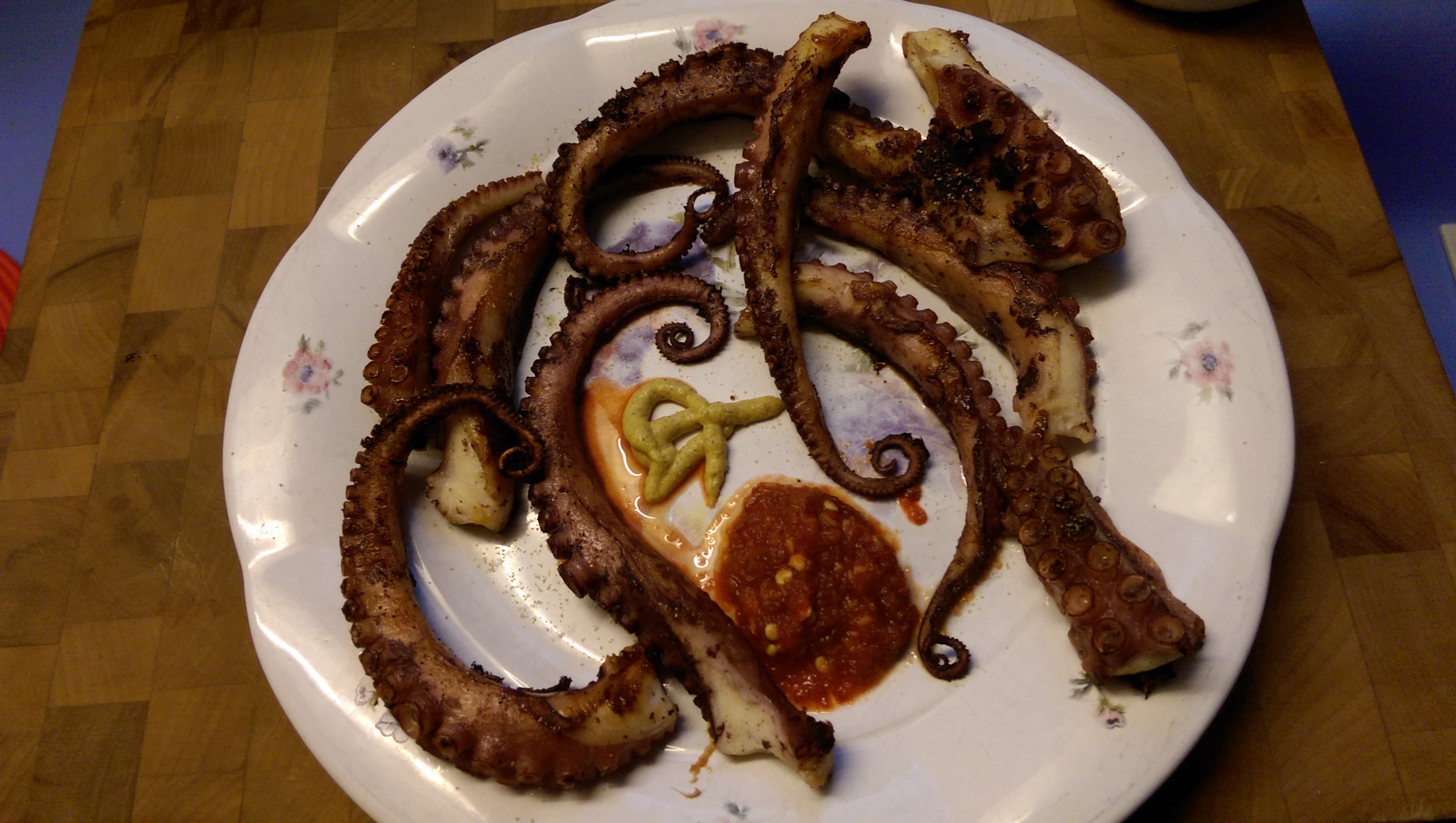This image depicts a wooden table composed of rectangular planks in varying shades of brown. The top left and right edges feature a purplish-blue background. At the center of the table sits a large white, ceramic dinner plate with gently scalloped edges, adorned with pink and purple floral designs. The plate holds several pieces of fried octopus, cooked to a deep golden brown, with their ends slightly curled. The pieces are sizable, suggesting they are whole sections of octopus arms. In the middle of the plate, there's a generous dollop of red cocktail sauce, complemented by a strip of mustard squeezed out of a tube.